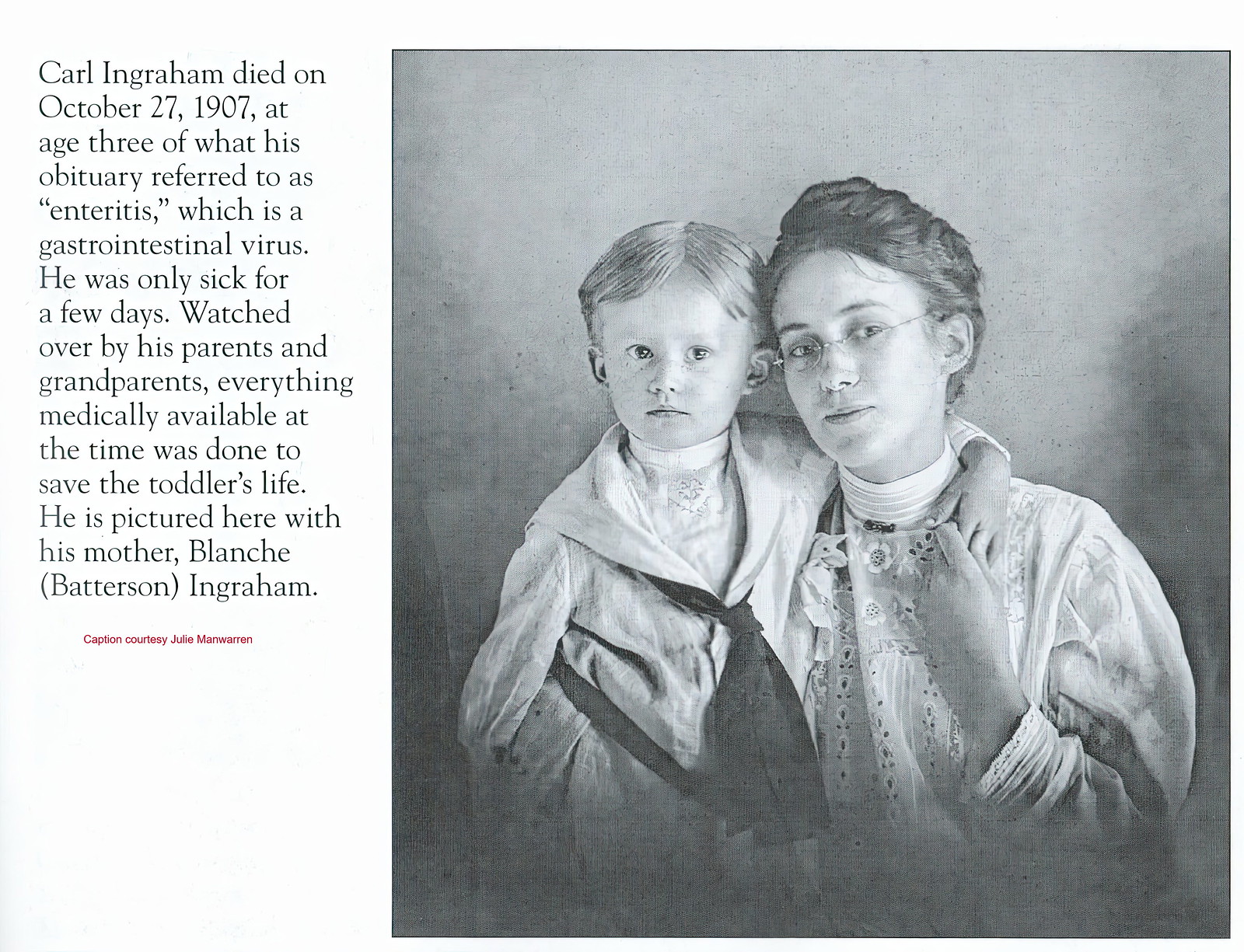The black-and-white photograph prominently positioned on the right side of the image features a poignant captured moment between a mother and her young son. The child, estimated to be around three to six years old, stands to the left of the woman, his right arm wrapped endearingly around her waist. He has short, center-parted blonde hair and is dressed in a sailor suit, complete with an ascot and delicate ruffles, topped off by a high, white collar that fully covers his neck. His face, though neutral, looks off to the right of the camera.

To the right of the boy stands his mother, identifiable as Blanche Batterson Ingraham, who is wearing a light-colored, frilly dress. Her hair is pinned up neatly in a bun, and she sports thin glasses. While her face shows a subtle smirk, there is a depth of emotion captured in her gaze. The backdrop of their photograph is an evenly lit, smooth gray, which darkens and fades at the bottom edges.

To the left of the photograph, the text provides a somber context to the image. It reads: "Carl Ingraham died on October 27, 1907, at age three, of what his obituary referred to as enteritis, a gastrointestinal virus. He was only sick for a few days, watched over by his parents and grandparents. Everything medically available at the time was done to save the toddler's life. He is pictured here with his mother Blanche (Batterson) Ingraham." The caption ends with a small credit in red letters, "Caption courtesy, Julie Manwarren."